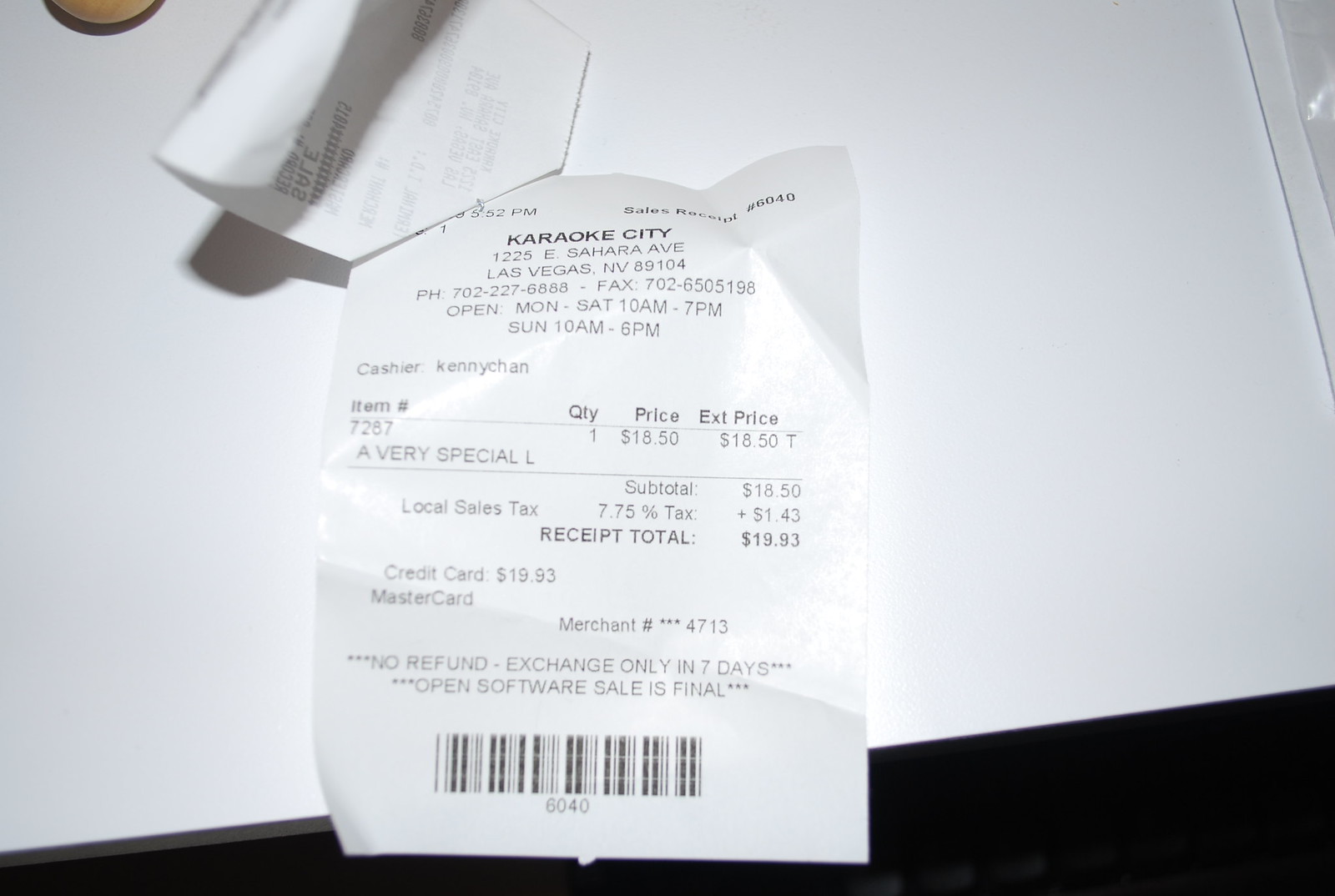Close-up photo of a wrinkled, thermal receipt stapled at the top left corner, lying on a white table surface. Partially obscured by a folded receipt facing away, the visible receipt is from Karaoke City, located at 1225 East Sahara Avenue, Las Vegas, Nevada, 89104. The receipt includes contact information and hours of operation. It details a purchase of a special L costing $18.50, with an added 7.75% sales tax of $1.43, culminating in a total of $19.93, paid via MasterCard. The merchant number is 4713, and the receipt notes a no-refund policy with exchanges allowed within 7 days.